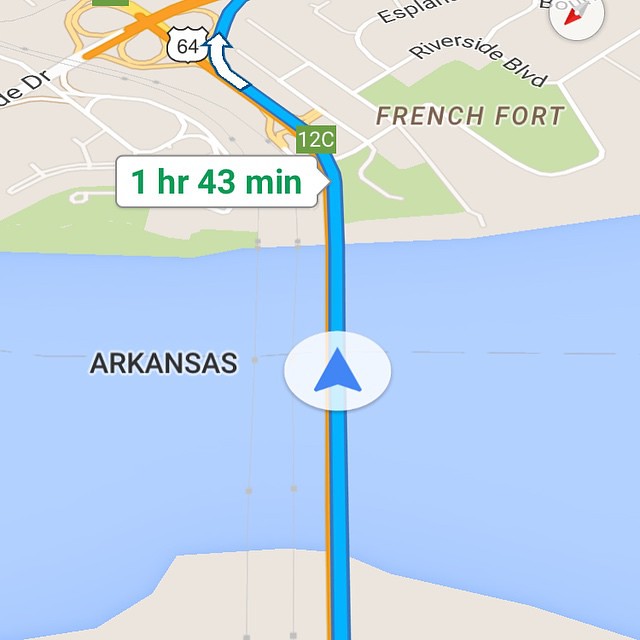This image displays a digital map of Arkansas on an electronic device. In the center-left portion of the map, the word "ARKANSAS" is prominently displayed in black capital letters. The lower section of the map is predominantly blue, suggesting it represents a body of water, and it transitions into a beige area towards the bottom. A blue line, indicative of a route, traverses this body of water, veering leftward and then slightly upward toward the top third of the map.

The upper third comprises a network of roads and land areas depicted in green and beige, with several curving roads and lines delineating the geography. An arrow inside a white circle is positioned in the middle of the blue section, pointing upward. Additionally, along the highlighted route in the upper area, there is a green quote bubble displaying the text "1 hour and 43 minutes." Various places and roads in the top part of the map are labeled with names, adding to the navigational detail.